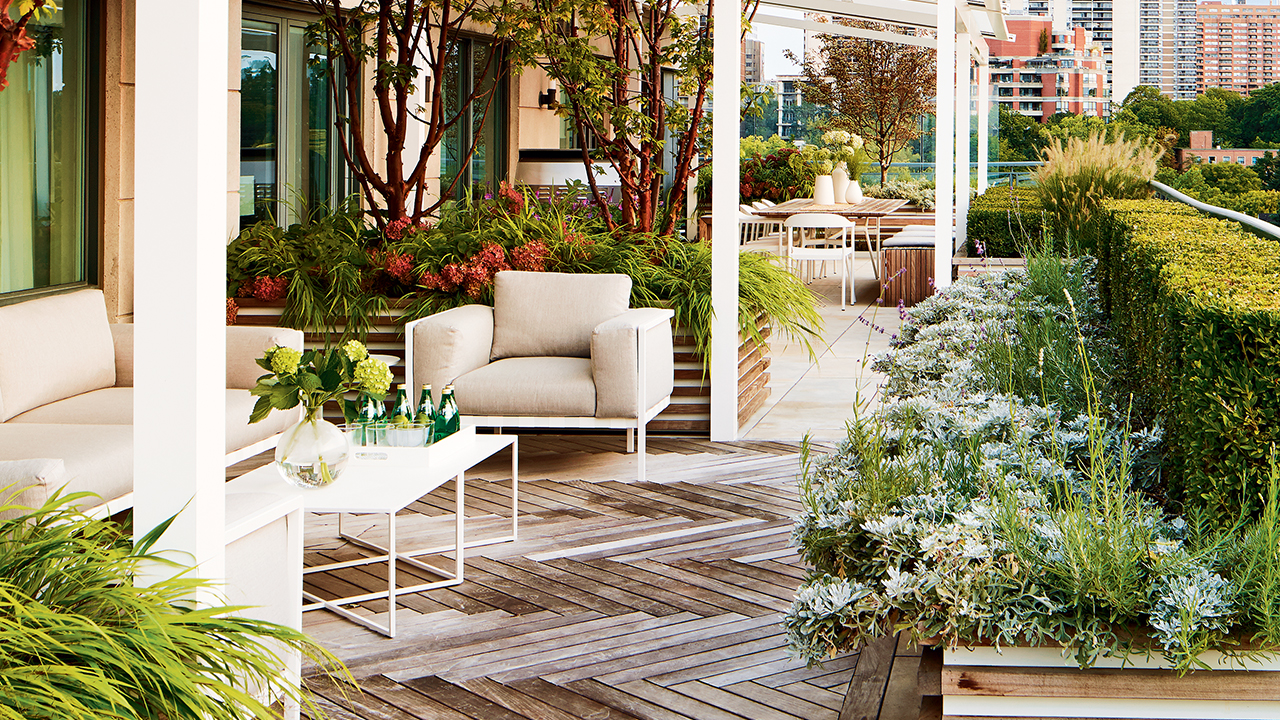The photograph captures a stylish rooftop patio with a brown wooden deck, abundant with greenery and cityscape views. A cozy seating area occupies the left side, featuring a two-seater outdoor couch and a matching single armchair, both adorned with tan cushions. Between these seats, a white-framed coffee table holds several green bottles with gold caps, presumably Perrier, and a round vase filled halfway with water and yellow flowers. Surrounding the seating arrangement, various planters host a vibrant mix of greenery, from white flowers and red blooms to square-cut hedgerows and small trees. Further into the scene, an outdoor dining table with white chairs and multiple vases of white flowers is visible. The backdrop showcases an array of towering city buildings, adding an urban touch to this tranquil garden-like space.